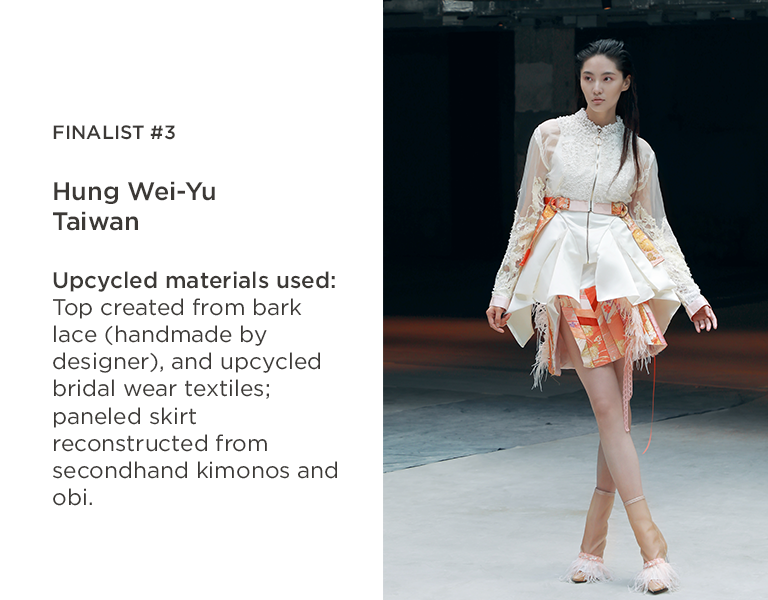The image features a young, slender Asian woman, likely a model, showcasing an intricate fashion piece as a finalist in a design competition. On the right side of the image, she is pictured in a striking pose, possibly on a runway with a gray concrete floor beneath her and a dark, indistinct background. She sports a dazzling white dress that comprises a combination of sheer and lacy fabrics. The dress has long, see-through sleeves adorned with embroidered details and a white lacy top. 

An orange belt cinches her waist, accentuating the dress's short, ruffled skirt, which ends above her knees. Beneath this outer layer, another skirt peeks out, featuring vibrant orange, red, and yellow floral patterns crafted from upcycled bridal textiles and secondhand kimono fabrics. Her footwear includes high-heeled shoes adorned with ruffled, lacy pink fabric near the toes, adding a whimsical touch to her ensemble. 

The left side of the graphic contains a textual description of the fashion piece, identifying the designer as Hung Wei Yu from Taiwan, finalist number three in the competition. The text highlights the use of upcycled materials, including a top made from bark lace and a paneled skirt reconstructed from secondhand kimonos and obi. The model's long black hair cascades behind her, completing her elegant look.